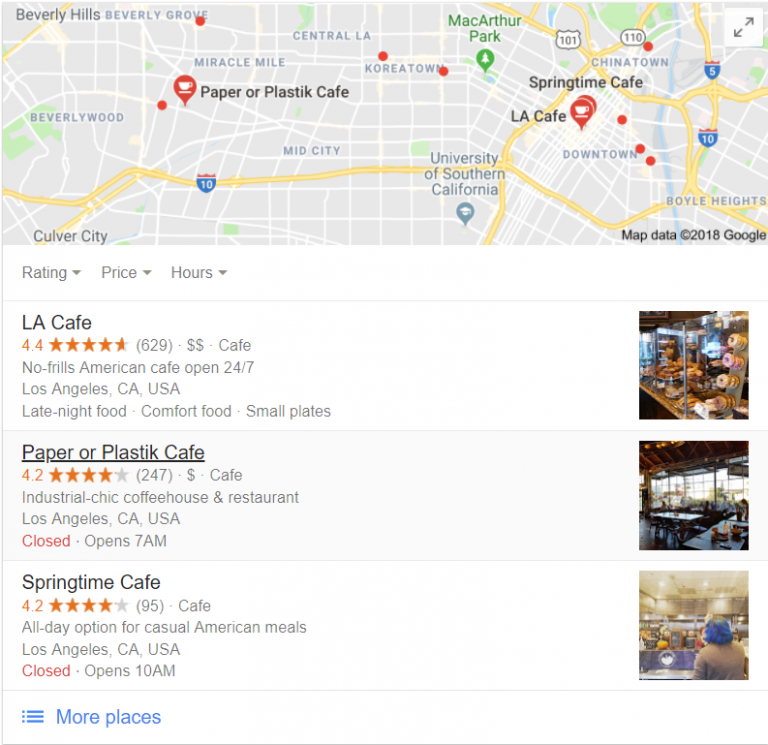The image is a screenshot of a map from a Google website, specifically depicting an area in Los Angeles, California. The map prominently shows various cafes and restaurants, indicating places to dine. In the top section, the map clarifies its source with the label "Map Data 2018 Google." 

Highlighted details include a yellow line representing a highway and white lines for smaller streets. Among the notable cafes marked on the map are LA Cafe, Paper or Plastic Cafe, and Springtime Cafe. Detailed information such as their ratings, average costs, and types of cuisines (primarily baked goods and coffee) accompanies these listings. The visual guidance provided to the right of the map suggests the offerings of each cafe.